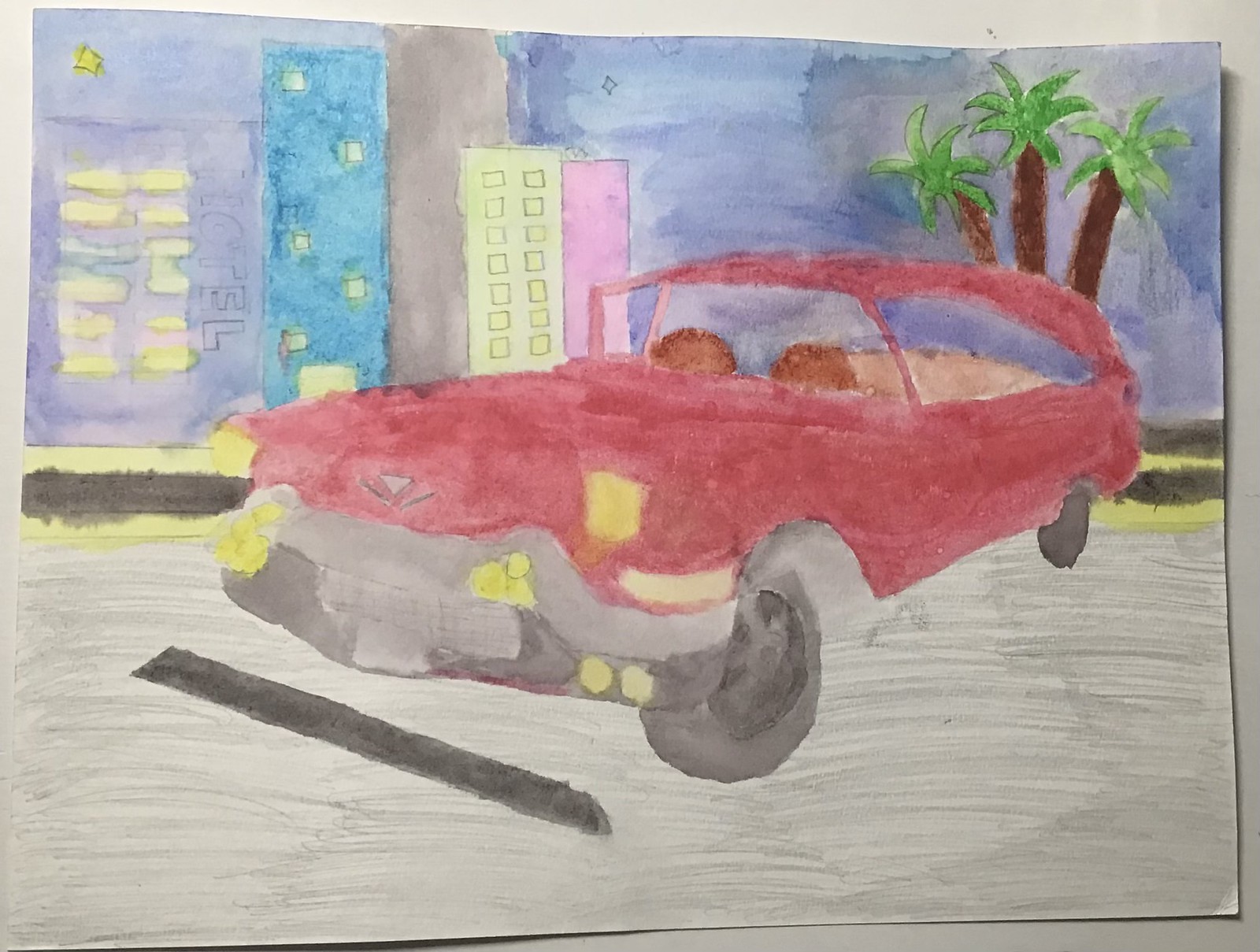This watercolor painting captures a vibrant red car prominently positioned in the center of the canvas, with its front hood facing forward and its back end angled slightly towards the right. The artist has skillfully blended watercolor techniques with pencil sketches and outlines, adding depth and detail to the composition. The car's clear windows reveal brown seats inside, while its left two wheels and silver bumper are depicted with meticulous attention to detail. The car's yellow headlights stand out against its red body, further enhancing its striking appearance. 

The scene is set in a gray parking lot, demarcated by a black bar indicating the parking spot in front of the car. The background features a lively mix of architecture and nature; three tall palm trees are grouped together, creating a sense of tropical ambiance. Various buildings painted in shades of purple, blue, gray, yellow, and pink add a splash of color to the backdrop, with one building distinctly labeled "hotel," indicating an urban setting. The entire composition blends elements of realism and artistic impression, resulting in a captivating and detailed depiction of a seemingly ordinary scene.